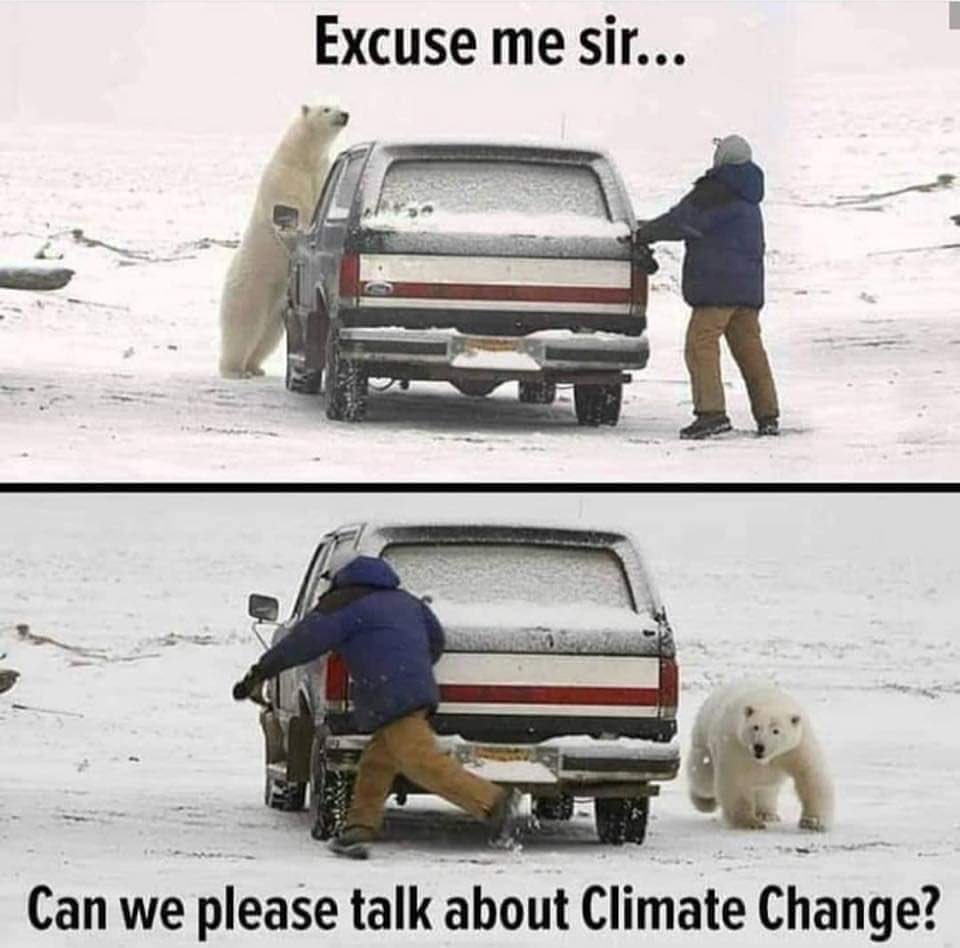In a snowy, flat landscape under cloudy skies, a meme unfolds across two images separated by a black line. The top image features a dark blue, older model Ford pickup truck with a gray and red tailgate, partially covered in snow. Black, sans-serif text at the top reads, "Excuse me sir...". To the right of the truck, a man in a navy blue coat, khaki pants, dark brown shoes, and a grayish cap stands with his hands on the truck bed. On the left side of the truck, a polar bear stands upright, staring at the man. The second image, slightly brighter in lighting, shows a dramatic turn of events. The polar bear has circled around the front of the truck and is now on all fours, in pursuit of the man who is retreating toward the left side of the truck in a run. The bottom caption in the same black sans-serif font reads, "Can we please talk about climate change?"